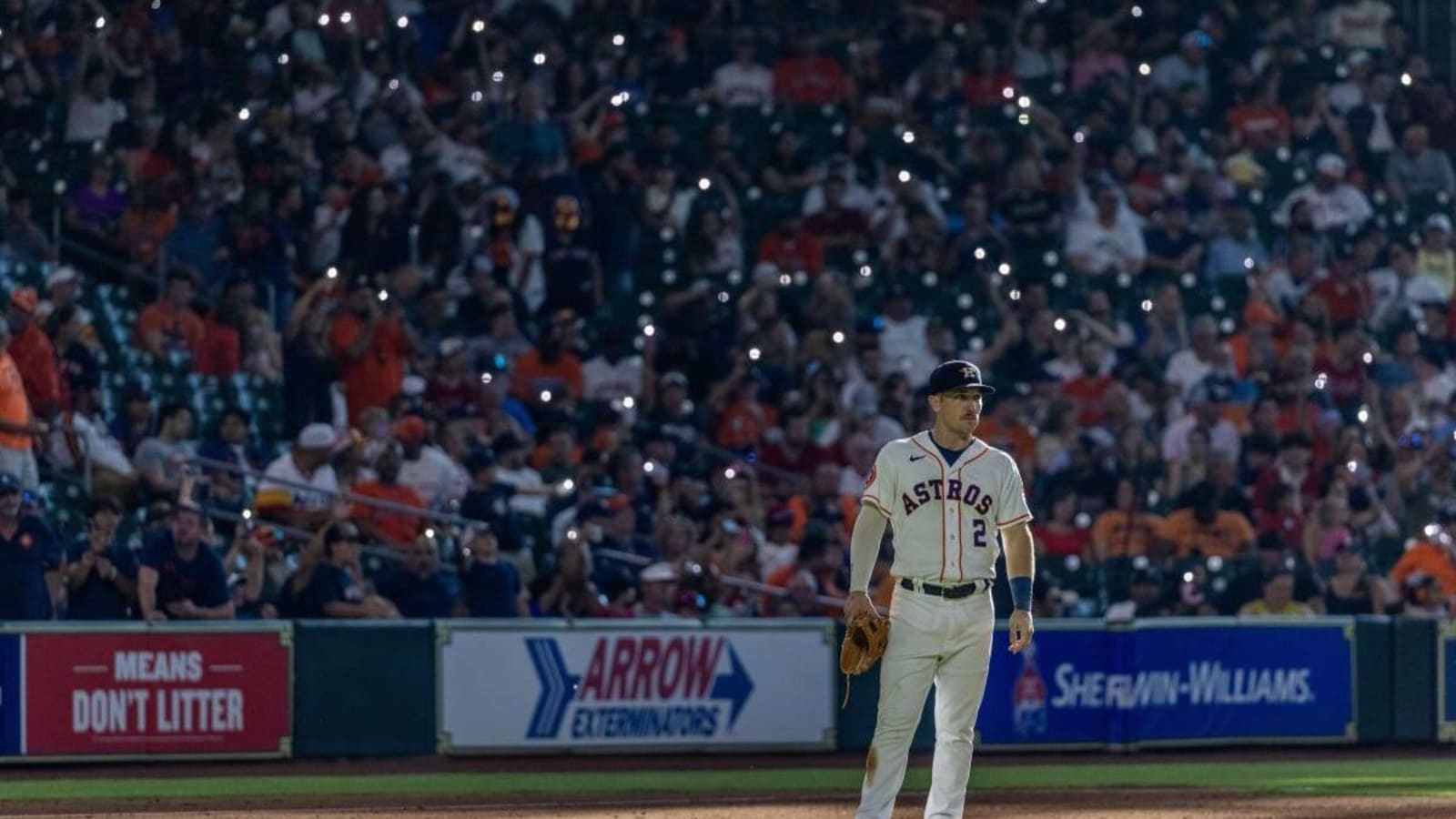This is a horizontal landscape photograph capturing a Major League Baseball player from the Houston Astros, wearing a white uniform with the number 2 and "Astros" emblazoned across the chest in orange trim. He stands slightly to the right of the center at the bottom of the frame on a brown dirt area with a green field visible behind him. His outfit includes a bluish hard cap and notable orange trimmings near the buttons, sleeves, and neckline. The player, likely a third baseman, holds his glove in his right hand while gazing towards the field.

In the background, the stadium crowd is visible but out of focus, adding to the dynamic atmosphere of the scene. Many spectators seem to be holding up lights, possibly from their mobile phones, giving an impression akin to a concert setting. Along the sides of the stadium, several banners are visible: one red sign advises not to litter, a white and blue one for "Arrow Exterminators" points with a stylized arrow, and a blue Sherwin-Williams logo emblazoned in white. The combined details and ambiance create a vivid portrait of a moment in a baseball game.